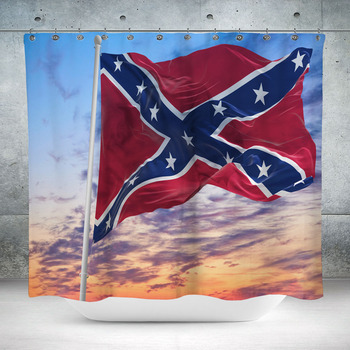The image shows a shower curtain depicting the Confederate flag. The Confederate flag features a red background with a large royal blue X outlined in white, and white stars are arrayed within the X. The shower curtain is suspended by gold hooks on a white pole. In the background, there is a dramatic sky with shades of blue, yellow, purple, and orange, resembling a sunset with dark clouds. The curtain is set against a bathroom scene, where part of a gray tile wall and the bottom of a white bathtub can be seen below the curtain.